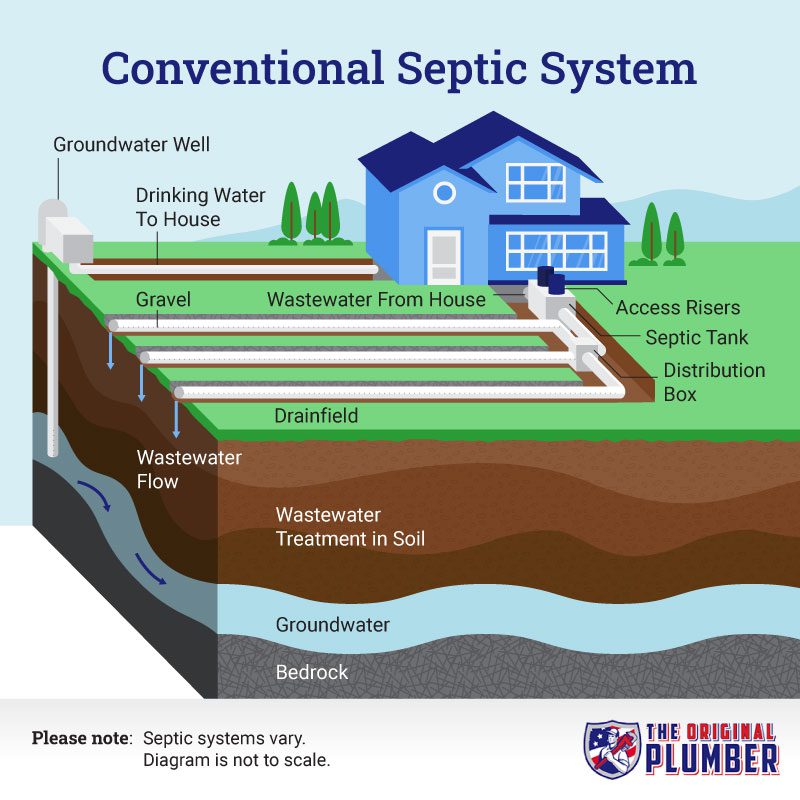This detailed diagram illustrates a conventional septic system. At the top, the title "Conventional Septic System" is prominently displayed in dark blue font. The central image is a clip-art styled illustration of a two-story blue house with a dark blue roof, white windows in the form of a circle and rectangle, and it's placed on a verdant field of grass with a couple of trees. The ground beneath the house is sectioned to reveal a comprehensive view of the septic system components.

In the layered cross-section of the ground, brown represents the soil layers, beneath which is light blue groundwater. Further down is a gray bedrock layer. Various parts of the septic system are annotated and labeled: it starts from the wastewater flowing from the house into a series of white tunnels and sewer drains, leading to a septic tank and then to a distribution box. From there, wastewater is directed to a gravel-filled drain field. Additional components like access risers, wastewater treatment, soil treatment, and the groundwater well are also highlighted. There’s a clear distinction between treated drinking water going into the house and wastewater being managed.

In the bottom left-hand corner, the diagram includes a note stating, "Please note this septic system diagram is not to scale." The bottom right-hand corner features "The Original Plumber" logo in red, white, and blue colors, representing the company responsible for the diagram.